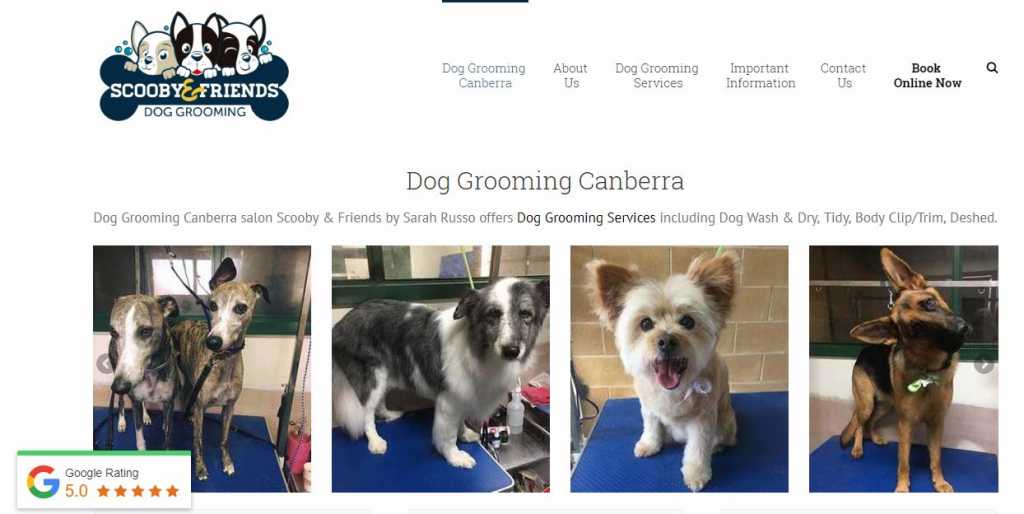Screenshot showcasing four images in a grid format, featuring three dogs in various poses. The screenshot is headed by a green bar containing navigation options such as "About Us," "Dog Grooming Services," "Important Information," and "Contact Us." Additionally, there's an option to "Look Online Now," accompanied by a magnifying glass icon.

The primary focus is on the dog grooming services offered by "Scooby and Friends Dog Grooming Salon" located in Canberra, owned by Sarah Russell. The services listed include dog wash and dry, tidy body clip/trim, and more. The images depict a variety of dogs: two brown and white, one black and white, and another with brown and black fur.

A "G" icon in Google colors is present, along with a 5.0-star rating and customer reviews symbolizing high satisfaction with their services.

The overall presentation emphasizes high-quality dog grooming services, detailed information about the offerings, and positive customer feedback, making it a compelling advertisement for potential clients.